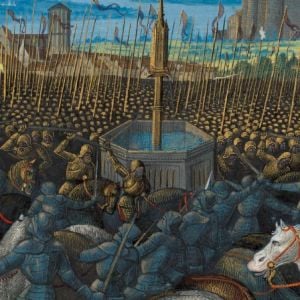The image vividly illustrates a medieval battle scene rendered in a stylized artistic format. Thousands of soldiers, primarily clad in gold armor, are depicted engaging in combat. The soldiers, predominantly carrying dark brown pikes, form massive, dense ranks illuminated by a setting sun, casting a warm glow on the scene. The battlefield features an octagon-shaped well at its center, crowned by a golden statue, where many of the soldiers are seen either surrounding or hiding near it. In the foreground, a striking white horse curiously gazes into the fray, surrounded by soldiers in dark grayish-blue attire, suggesting a different faction in the conflict. The tumultuous scene is framed by a darkening blue sky, a castle wall to the left, and a towering mountain to the right, adding a sense of depth and grandeur to the painting. The overall impression is one of chaos and intensity, captured under the waning light of day.